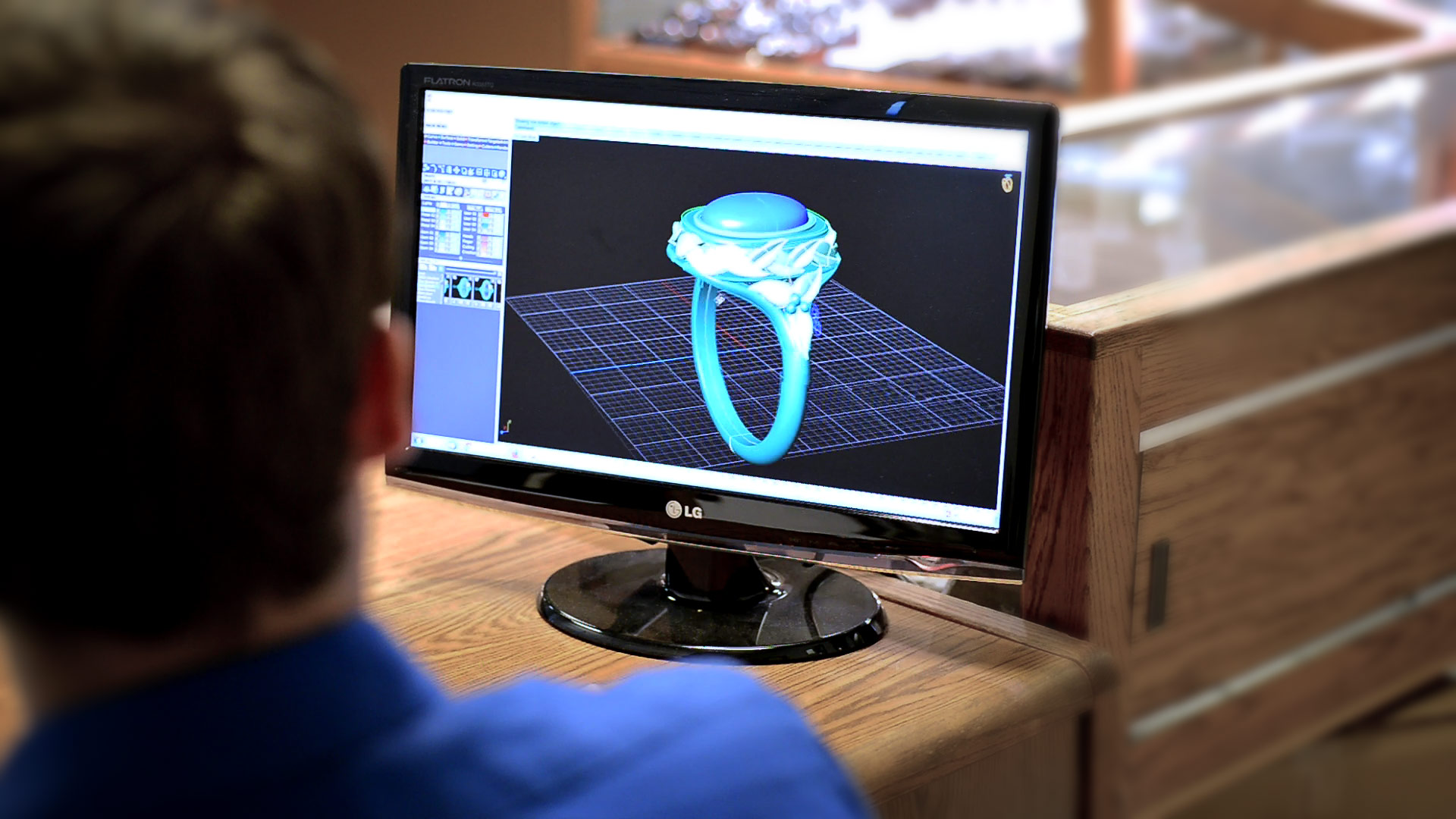The photograph captures a scene from behind a man with dark brown hair wearing a collared blue shirt. He’s seated at a wooden desk, his attention focused on an LG computer screen in front of him. The computer, trimmed in black, prominently displays a detailed, digitally-rendered image of a ring. The ring features an oval-shaped gemstone of a light blue hue, set against a black background with a silver-and-black mat at the bottom. The ring appears large, occupying almost the entire screen, which also shows a grid beneath the ring, indicating the use of a design program likely for jewelry making. The remainder of the background is blurred, emphasizing the focus on the computerized ring design.